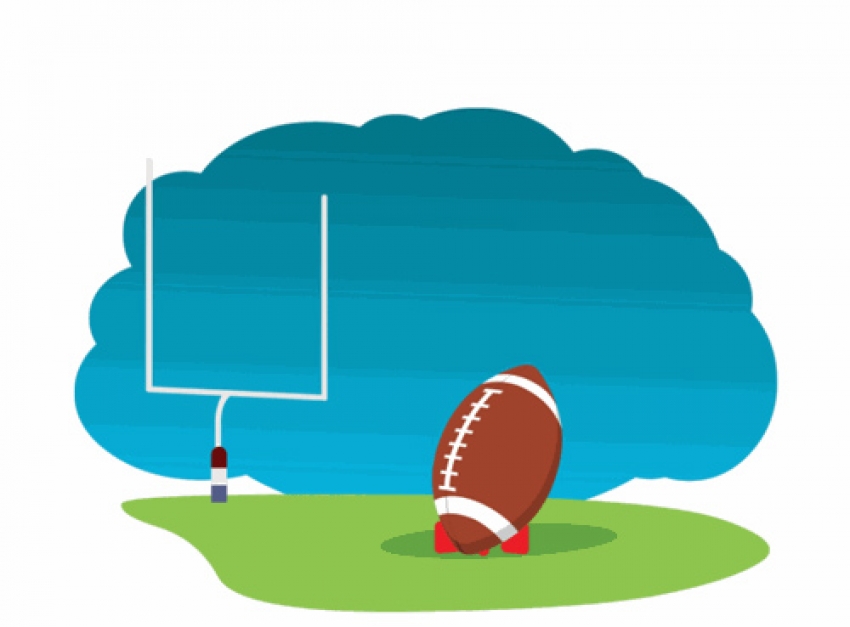The cartoon-like image portrays a simplistic scene of an American football field that appears to be computer-generated or reminiscent of old clipart. Dominating the foreground is a brown football, detailed with bold white trims in the middle and solid white trims at the top and bottom, resting on a red kickstand, casting a shadow on the grass beneath it. The green splotch of grass, devoid of any yard lines, extends back to an American football goal post in the background. The goal post features a U-shape with red, white, and blue trims at the bottom. Above all, the backdrop transitions from a deep to a light blue, representing the sky, capped by a massive, blue cloud shape. The setting is distinctly outdoors, meant to depict a basic yet recognizable sports clipart of a football setup.